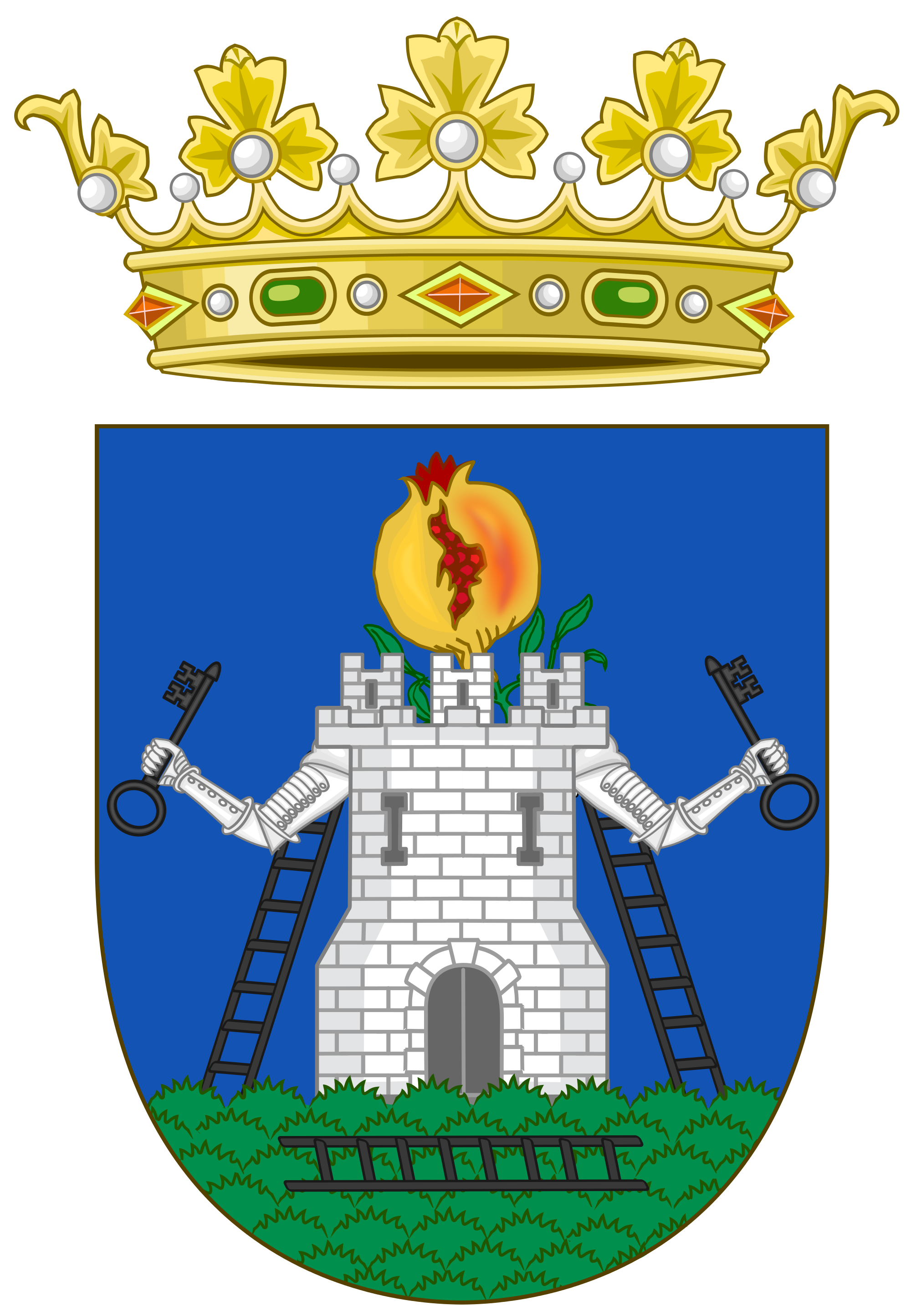This detailed, digitally illustrated royal emblem features a crown and a crest, set against a white background. The crown is goldish-yellow and adorned with red and green jewels, white pearls, and intricate gold leaves each topped with a pearl. Beneath this vibrant crown lies a shield-shaped crest with a blue backdrop. The central figure of the crest is a white castle, flanked by green bushes, and adorned with two human-like arms emerging from its sides, each holding a large black key. Above the castle's turret, a flower-like object resembling a yellow and red pomegranate bursts with life. Three ladders are present: two leaning against the castle and one horizontally placed in front of the green shrubs. The entire scene exudes a hand-drawn, cartoonish charm while maintaining the traditional intricacy of a royal emblem.